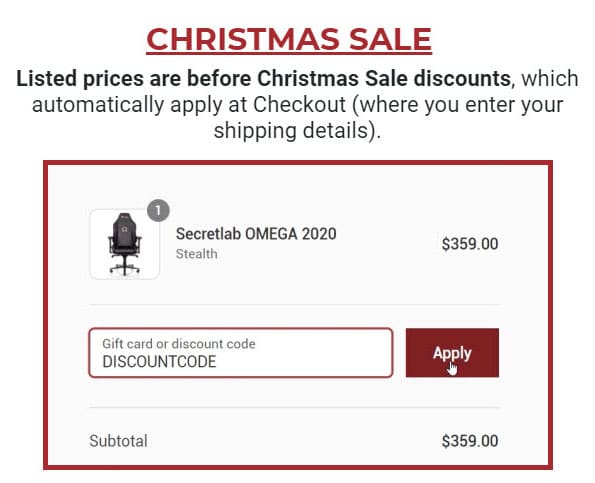The website displayed resembles an Amazon-style online store, prominently featuring a "Christmas Sale" announcement in bold red letters at the top. Just beneath, in black text, it notes: "Listed prices are before Christmas sale discounts, which automatically apply at checkout, where you enter your shipping details."

The main section showcases a product on the left, specifically a "Secret Lab Omega 2020" computer chair, tagged with the color "Stealth" in gray text. Next to the product image, the price is clearly marked as $359.00. Beneath the product listing, instructions for using a gift card or discount code are provided in black lettering, accompanied by a large red box labeled "Discount Code" and a red "Apply" button in white text.

At the bottom of this section, the "Subtotal" is displayed in black text with a corresponding price of $359.00 to the left. Overall, the website highlights a special holiday promotion with clear information and instructions for potential purchasers.